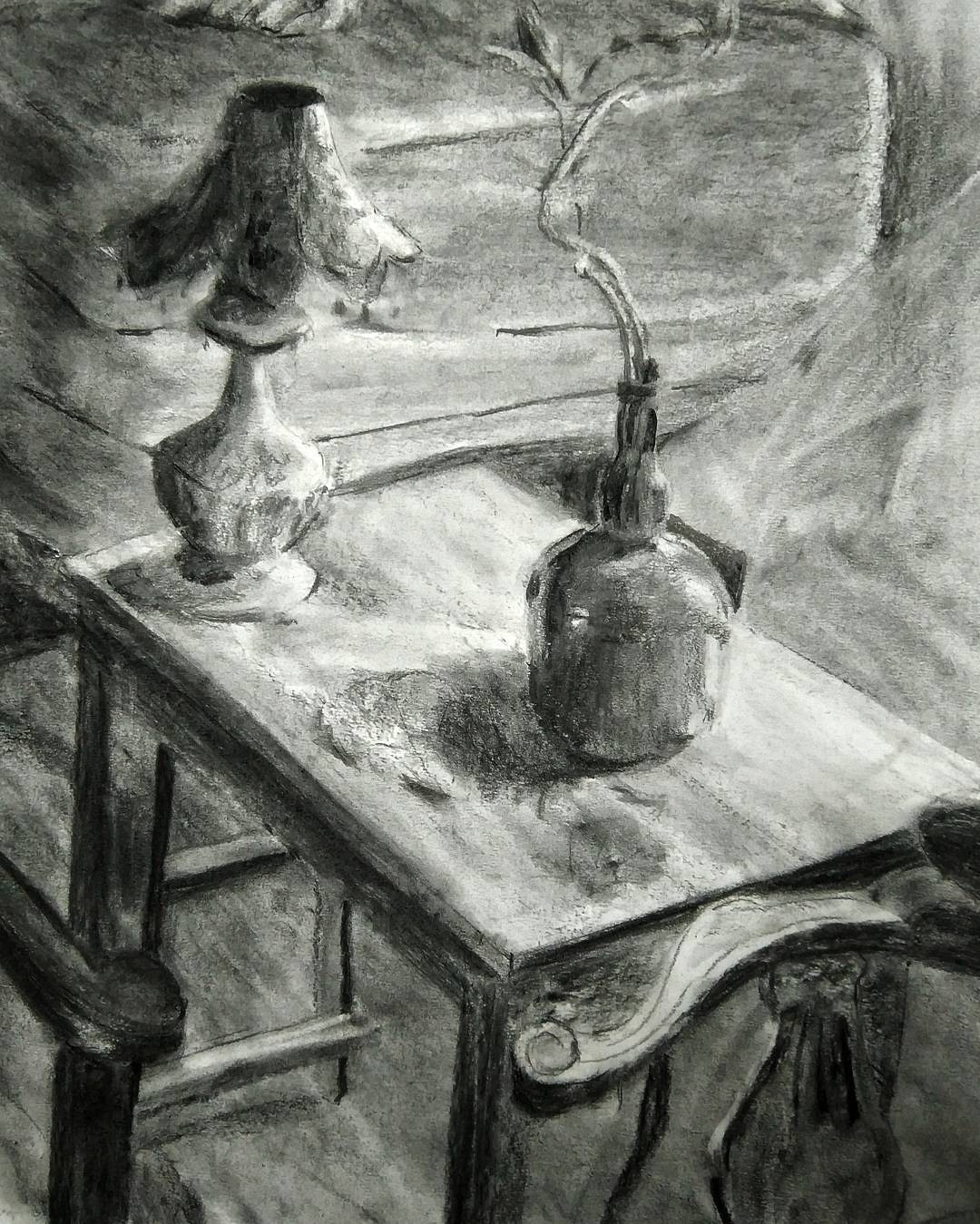This is a black and white illustration, possibly drawn with pencil or charcoal, showcasing a highly detailed, portrait-shaped scene. At the center is an ornate, rectangular table with a curved front edge. Resting on the table is an oval-shaped vase from which a narrow, winding stem with abstract flowers or buds emerges. The vase casts a shadow and might be placed on a placemat. In the upper left corner, a table lamp with a round base that tapers to a narrow neck is adorned with a feminine-looking, upside-down petal-shaped lampshade. The intricate design extends to the right-hand side and leg of the table. A hint of a wooden chair’s arm peeks into the frame on the right. In the background, a stack of cushions is visible, shaded lightly with pencil. The wall and floor exhibit significant shading, contributing to the depth and texture of the artwork, yet the upper right-hand corner remains simply shaded without detailed elements. The absence of text keeps the focus on the meticulously drawn elements of this artwork.